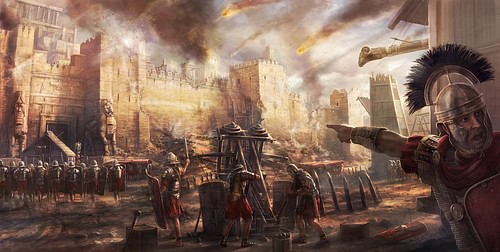The image depicts an intense battle scene, rendered in the style of an oil painting, set during a dramatic sunset or sunrise. The setting suggests an ancient Roman siege, characterized by a walled city or a large beige castle in the background, which appears to be under a heavy attack. Flaming projectiles and cannon fire are visible in the sky, likely launched from catapults and ballistae operated by Roman soldiers.

In the foreground on the right side, a Roman soldier, distinctively clad in red and metallic armor with a feathered helmet, is pointing towards the besieged castle. His gesture directs the attention of his comrades, who are gathered around siege towers and preparing for the attack. The soldiers, identified as Roman legionaries by their large shields and gladii (short swords), exhibit a determined readiness for battle. The city, engulfed in flames and thick smoke, vividly illustrates the chaos and ferocity of the conflict.